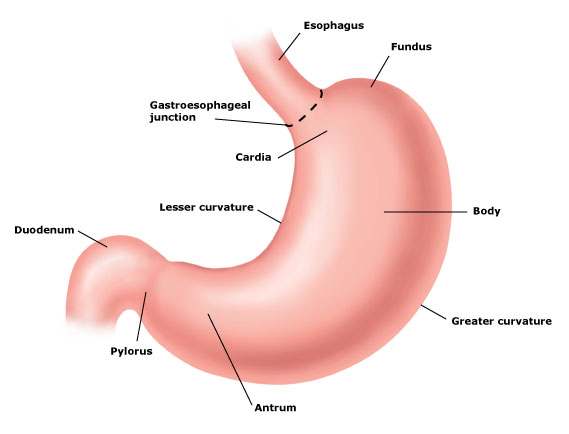This detailed, educational diagram illustrates the human stomach and its related organs, set against a completely white background. Central to the image is a pink-shaded stomach, meticulously labeled with black text to identify each component. From top to bottom, the diagram starts with the esophagus leading into the gastroesophageal junction and fundus at the top portion. Below these are the cardia and the central body of the stomach. The left side of the stomach features the lesser curvature while the longer, right side showcases the greater curvature. Moving downwards, the bottom left of the stomach is labeled as the antrum, progressing to the pylorus, and finally connecting to the duodenum on the far left. The image resembles a page from a medical textbook, emphasizing a clear and instructive presentation for educational purposes, complete with structure and function labels surrounding the stomach for detailed reference.